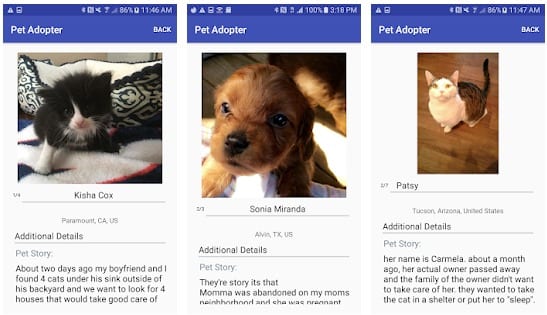Here are three detailed captions for the images, refined and cleaned up:

1. **Keisha Cox, Paramount, California**:
   A screenshot from the Pet Adopter app featuring a black and white kitten named Keisha Cox. According to the post, this adorable kitten was one of four found under an outdoor sink in someone's backyard. The finder is seeking loving homes for all four kittens. The first part of the detailed pet story mentions the discovery by the boyfriend of the poster, but the story cuts off after a few sentences.

2. **Sonia Miranda, Alvin, Texas**:
   This screenshot showcases a dog named Sonia Miranda, located in Alvin, Texas, as seen on the Pet Adopter app. The additional details section begins to tell the poignant story of Sonia's mother, who was abandoned in a neighborhood while pregnant. Unfortunately, the post is cut short, leaving out further details about Sonia's current situation and needs.

3. **Patsy (also referred to as Carmilla), Tucson, Arizona**:
   The third screenshot presents a cat named Patsy, also referred to as Carmilla, from Tucson, Arizona, on the Pet Adopter app. The pet story reveals that this cat's original owner passed away about a month ago, and the family did not want to take responsibility for her. The family had considered putting her to sleep or surrendering her to a shelter, with "sleep" notably placed in quotes. The full narrative is not available as the post is truncated.